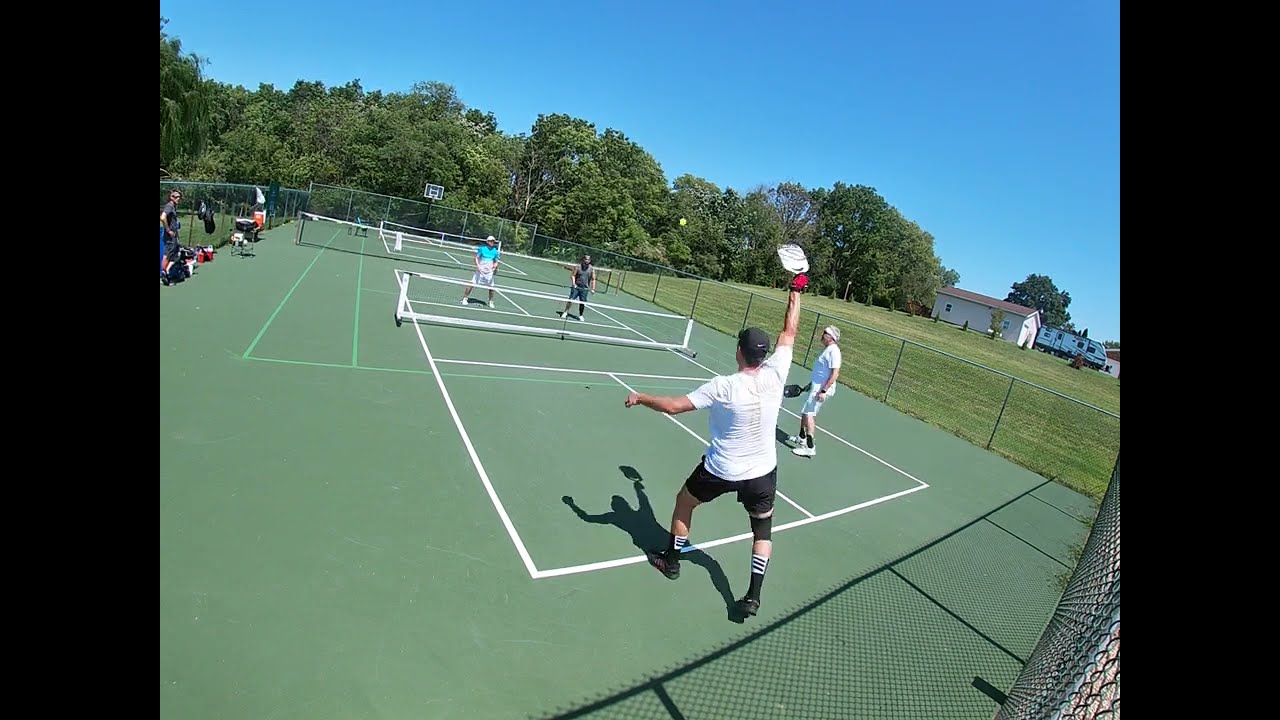In this color photograph, presented in landscape orientation with vertical black bars on both sides, an intense pickleball match unfolds on a dark olive green court marked with white lines. The court is surrounded by a chain-link fence, beyond which lies a recently mowed grassy field. On the far end of the field, a white wood-frame, one-story building is visible, accompanied by a motorhome. The horizon is lined with trees beneath a clear blue sky.

In the foreground, the pickleball action is captured with four men engaged in the game. The central figure closest to the viewer, poised to strike a greenish-yellow ball mid-air, sports a red glove on his right hand, a white shirt, black shorts, sneakers, and a black ball cap. Nearby, an onlooker in a white shirt and shorts stands attentively. The opposing team, also dressed in t-shirts and shorts, is poised to react on the other side of the net.

To the left, several individuals wait near the fence, ready to take their turn on the court. The composition and representational realism of the photograph suggest it was taken from a higher vantage point, possibly a drone, encapsulating the vibrant energy and detailed environment of the pickleball game.